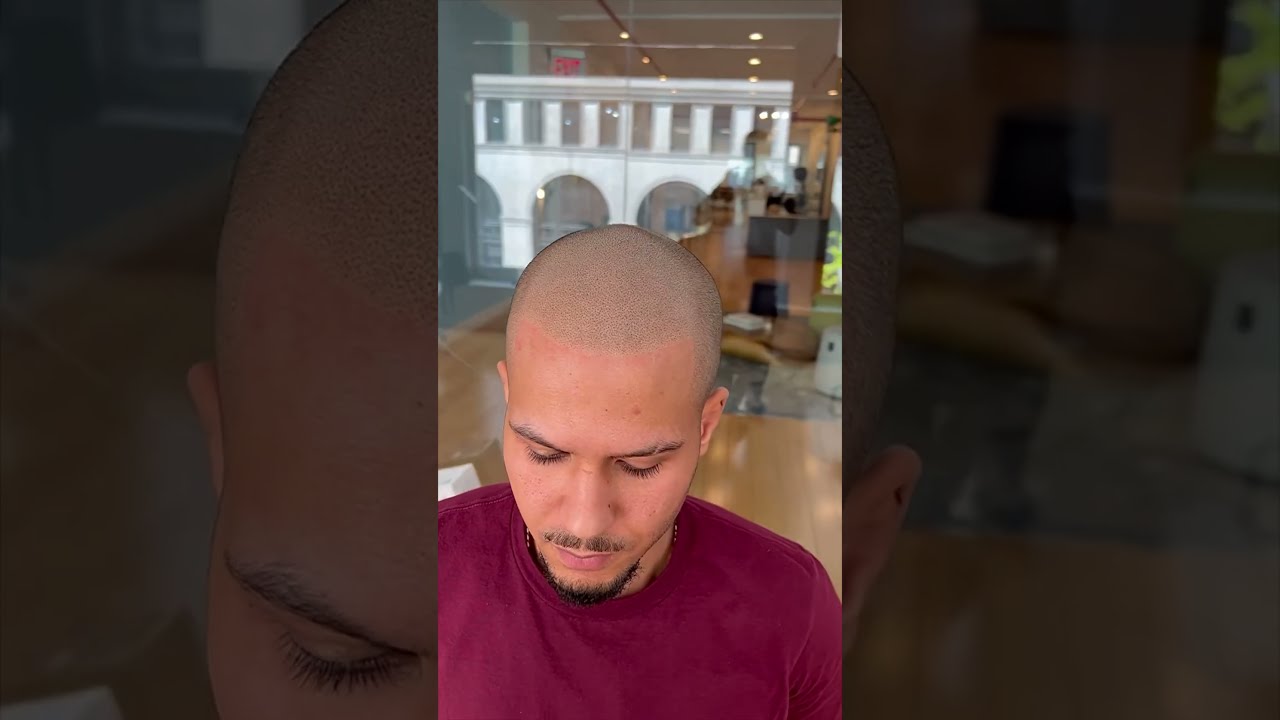In the image, we see a man in his late 20s with a buzz cut, giving him an almost bald appearance due to his very short black hair. He has a mustache and a goatee, the beard lining the edge of his chin and bottom lip. The man is wearing a dark red or maroon t-shirt and is shown from the armpits up. He is looking down, and although his eyes aren't visible, his eyebrows suggest a frown, and his eyes are possibly closed. The perspective of the photo is slightly elevated, capturing the top of his head and his downward gaze.

The background of the image shows a shiny light wood floor and what appears to be a see-through glass wall or doors leading to another section of the building. Reflections in the glass suggest it's daytime, with hints of the outside environment. Behind the glass, there are brown pillows and a brown table, hinting at an interior space that could be part of a store, an office, or perhaps an art gallery. The image itself is framed by a vertical cell phone picture style with faded, zoomed-in versions of the same image on either side, creating a gradient border effect.